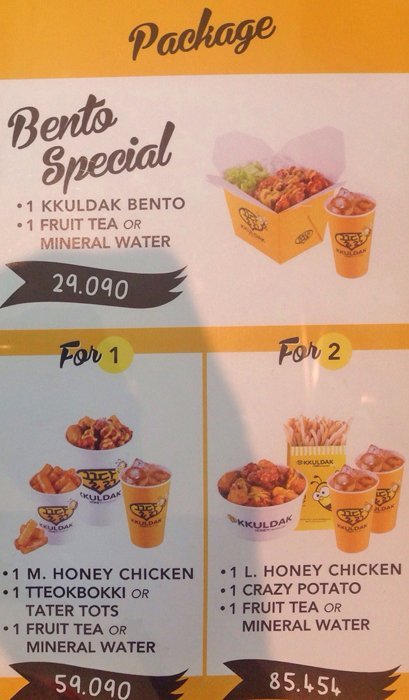The image presents a detailed menu for a restaurant offering various meal packages, likely not located in America and specializing in chicken dishes. At the top, prominently displayed against a yellow background, is the "Bento Special," which includes one Kuldak bento and a choice of one fruit tea or mineral water, priced at 29.090. The background for the price is a distinct black wavy banner. The advertised bento meal is depicted in a yellow, Chinese takeout-style box with a cup of tea next to it. Beneath this, the menu introduces two additional combo meals. The option "For One" includes one M honey chicken, a choice of teak baki or tater tots, and one fruit tea or mineral water, priced at 59.090. The "For Two" combo meal features one L honey chicken, a serving of crazy potatoes, and one fruit tea or mineral water, priced at 85.454. Packaging for the meals is characterized by bee-themed designs, and the establishment's name, "Cool Dock," appears prominently.